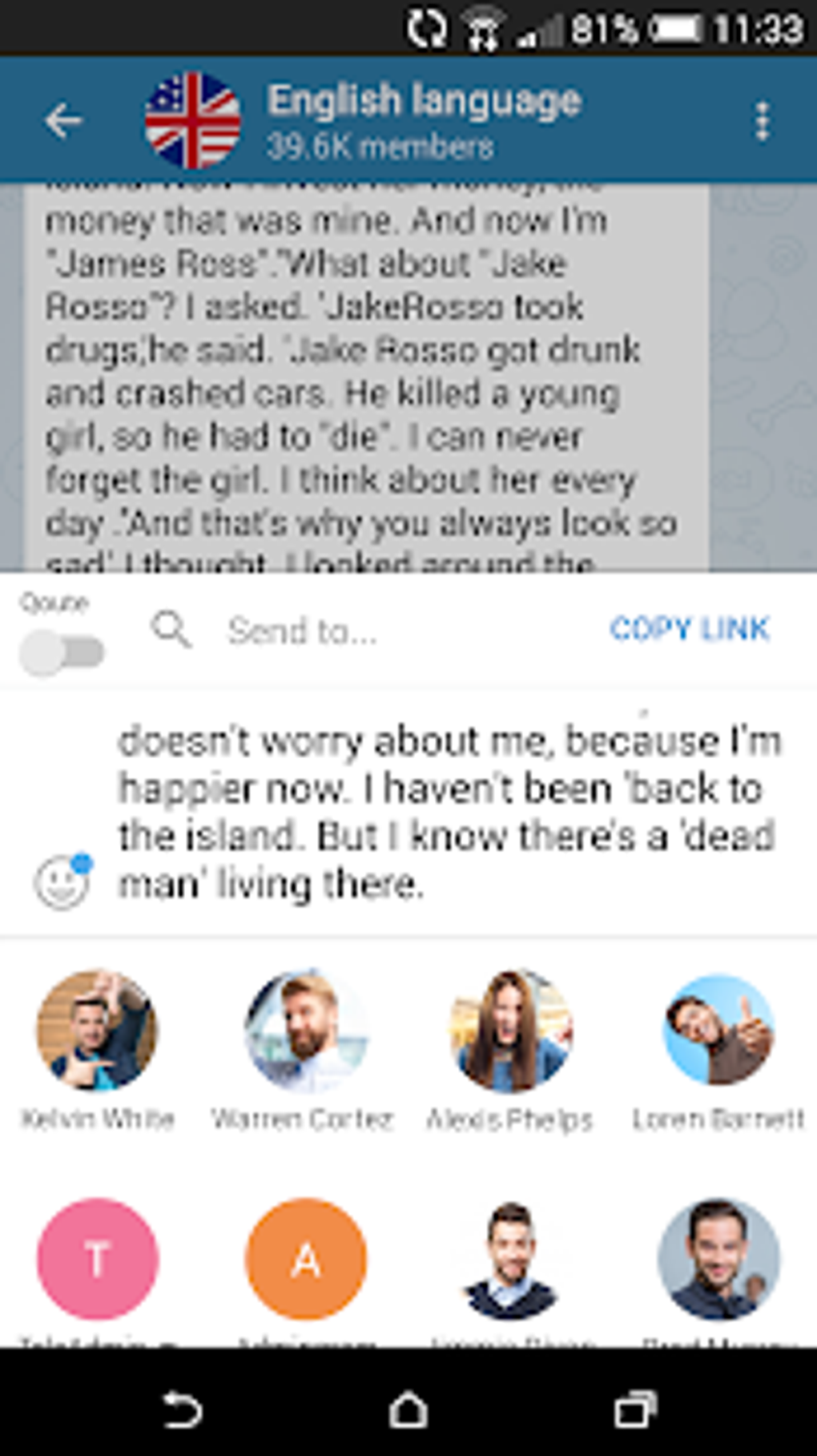This is a detailed screenshot from a mobile phone, displayed in portrait orientation with dimensions approximately twice as tall as it is wide. The top section features a horizontal black status bar containing several white icons. From left to right, these icons include a refresh symbol, a Wi-Fi signal at less than half strength, a network connection with two out of five bars, the battery percentage reading 81%, a horizontally oriented battery icon showing a white fill level, and the time displayed as 11:33.

Beneath the status bar, there is a prominent rectangular blue border housing a white left arrow, followed by a flag icon. This flag appears to be a composite of various English-speaking nations' flags with a red cross in the center. Beside the flag, the text "English language, 39.6 thousand members," is displayed, accompanied by a white speech bubble indicating a conversation or chat function.

The content section below this features a white box containing three interactive elements: a 'Send to search' button, a 'Copy link' button, and a block of black text that ominously states, "don't worry about me because I'm happier now. I haven't been back to the island but I know that there's a dead man living there."

At the bottom of the screenshot, there are four columns and two rows of avatars, totaling eight avatars. Six of these avatars display pictures, while the remaining two are represented by simple colored circles (one pink and one orange) each with a white letter in the center.